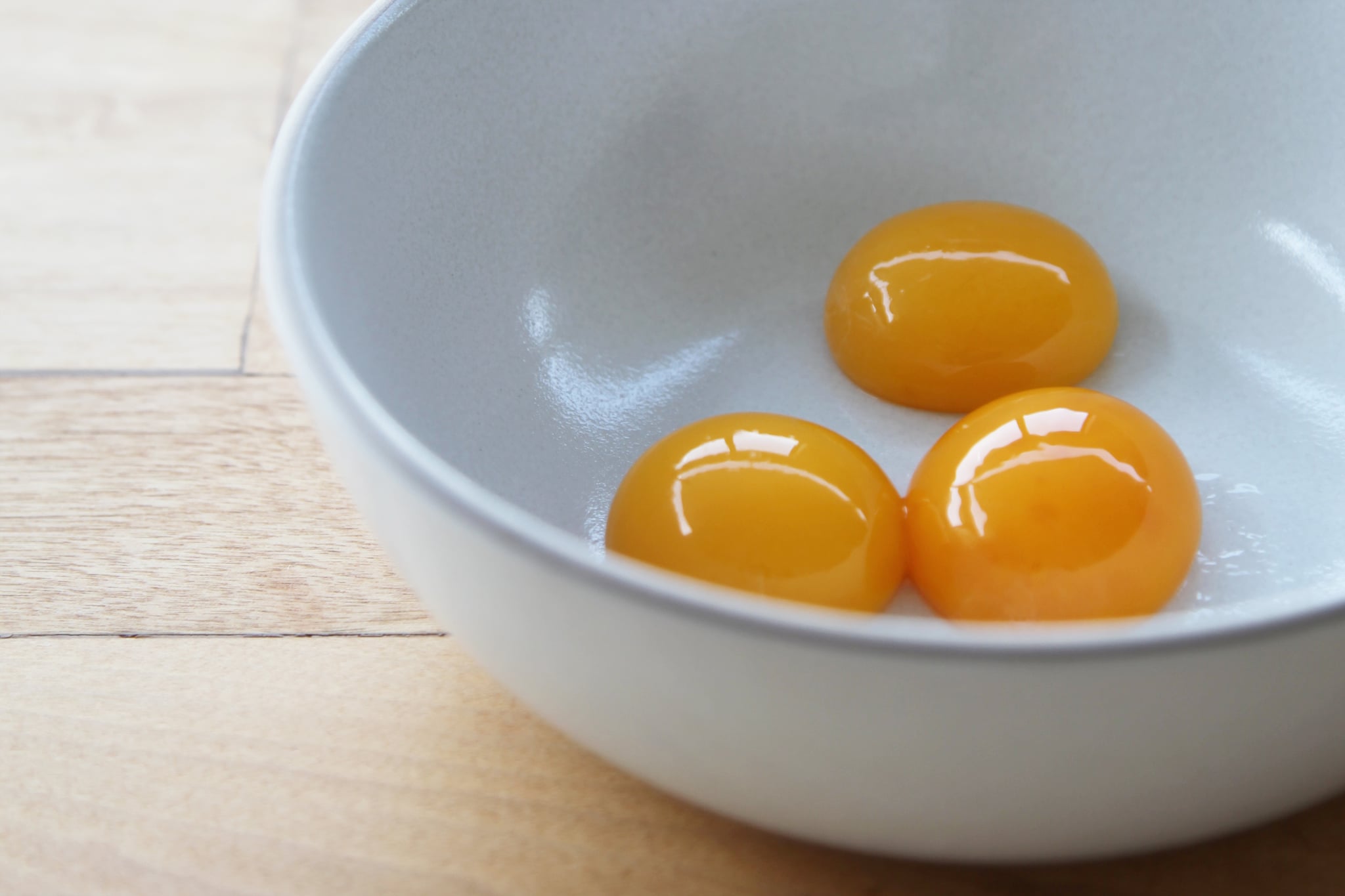The image captures a pristine, white, shiny ceramic bowl positioned towards the right side of the frame, partially cropped at its top right corner. Inside the bowl, three perfectly round, bright yellow egg yolks glisten under natural light, appearing almost dome-shaped with a reflective surface. Surrounding the yolks is a slight amount of clear liquid, suggesting minimal egg white. The bowl rests on a clean wooden surface comprised of variously oriented wood panels - some horizontal, some vertical, and some forming square shapes. The setting, likely a kitchen, is brightly lit, emphasizing the cleanliness and careful arrangement of the scene.